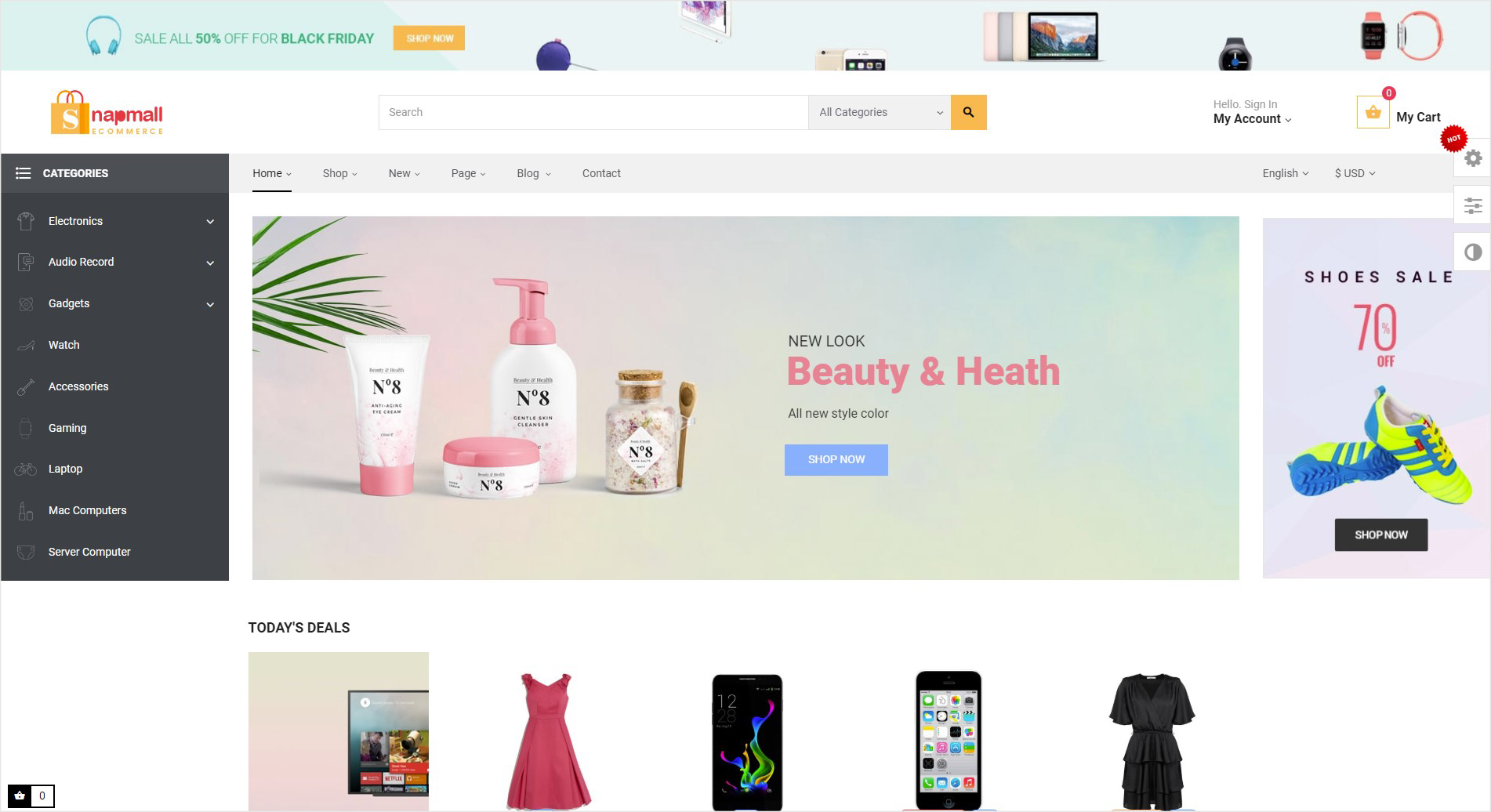This image is from the SnapMall website's homepage, prominently featuring a Black Friday sale with 50% off on all items. The top navigation bar is black and showcases the sale announcement in a central position, flanked by a pair of headphones on the left and a "Shop Now" button on the right. Beneath this bar, the SnapMall logo is displayed, combining a yellow shopping bag containing the letter "S" with "NapMall" in red text, and the word "e-commerce" underneath.

Adjacent to the logo on the same horizontal plane is a centrally justified search bar. On the left sidebar under the SnapMall logo, there's a vertical menu labeled "Categories," listing various product types including Electronics, Audio Record, Gadgets, Watches, Accessories, Gaming, Laptops, Mac Computers, and Server Computers. 

On the right-hand side, occupying the main window, is another vertical menu with navigation options: Home, Shop, New, Page, Blog, and Contact.